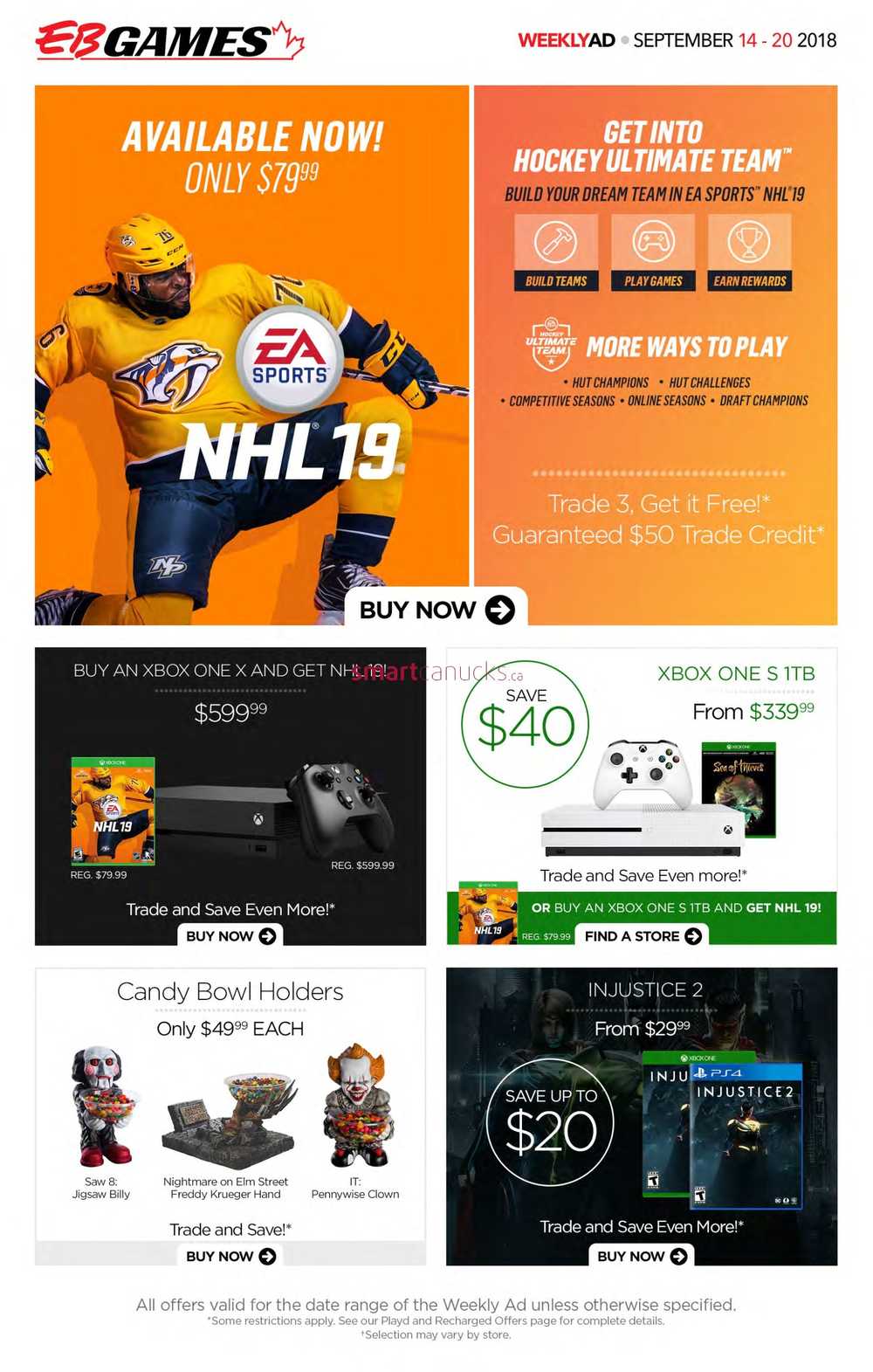This image showcases a screenshot of a landing page from EB Games, with a predominantly orange top section that is divided into two segments. The left segment features a promotional banner indicating that NHL 19 is "Available Now" for $79. This banner includes an image of a hockey player in a yellow uniform. Next to this, text encourages users to "Get in to Hockey Ultimate Team," highlighting three areas with "more ways to play." These sections are written in white text, separated by dotted lines and black borders. Additionally, it promotes a special offer: "Trade 3, get in free. Guaranteed," accompanied by a "Buy Now" button.

Below the orange banner, there are two lower blocks. The first block is black, displaying the NHL game alongside an Xbox console priced at $599. The adjacent block is white, featuring a similar Xbox console with the video game, but priced at $399. Beneath these blocks, there are candy holders, and next to them, a promotion for two Injustice video games.